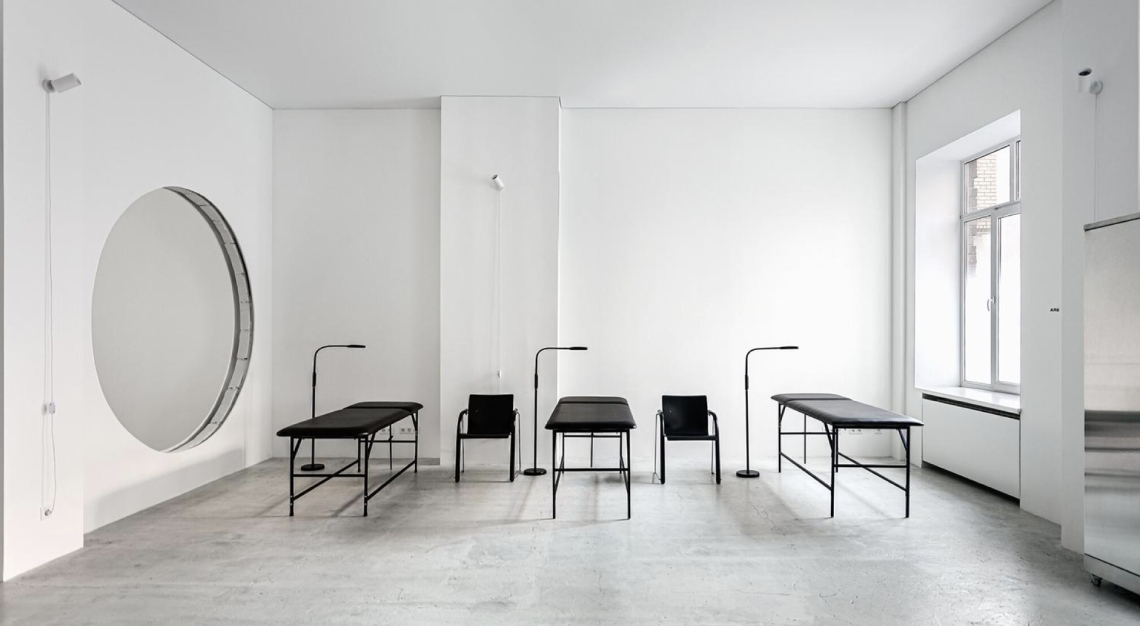This is a highly clinical and modern-looking white room with a stark, minimalist design. The room features white walls, ceiling, and grayish-white tile floors. Along the length of the room are three black examination tables arranged in a row, with two black chairs spaced in between them. Each table is illuminated by a gooseneck-style floor lamp bent toward the right. Light streams in through a deep-set window on the right wall, which has a three-panel design with a sliding panel at the top. The left wall features a large circular cutout that might be a window or mirror, though it lacks a visible reflection. In the foreground on the right side, a reflective stainless steel refrigerator door is partially visible, adding to the room's modern aesthetic. Suspended around the room are what appear to be lights or cameras, further emphasizing the room's clinical purpose.